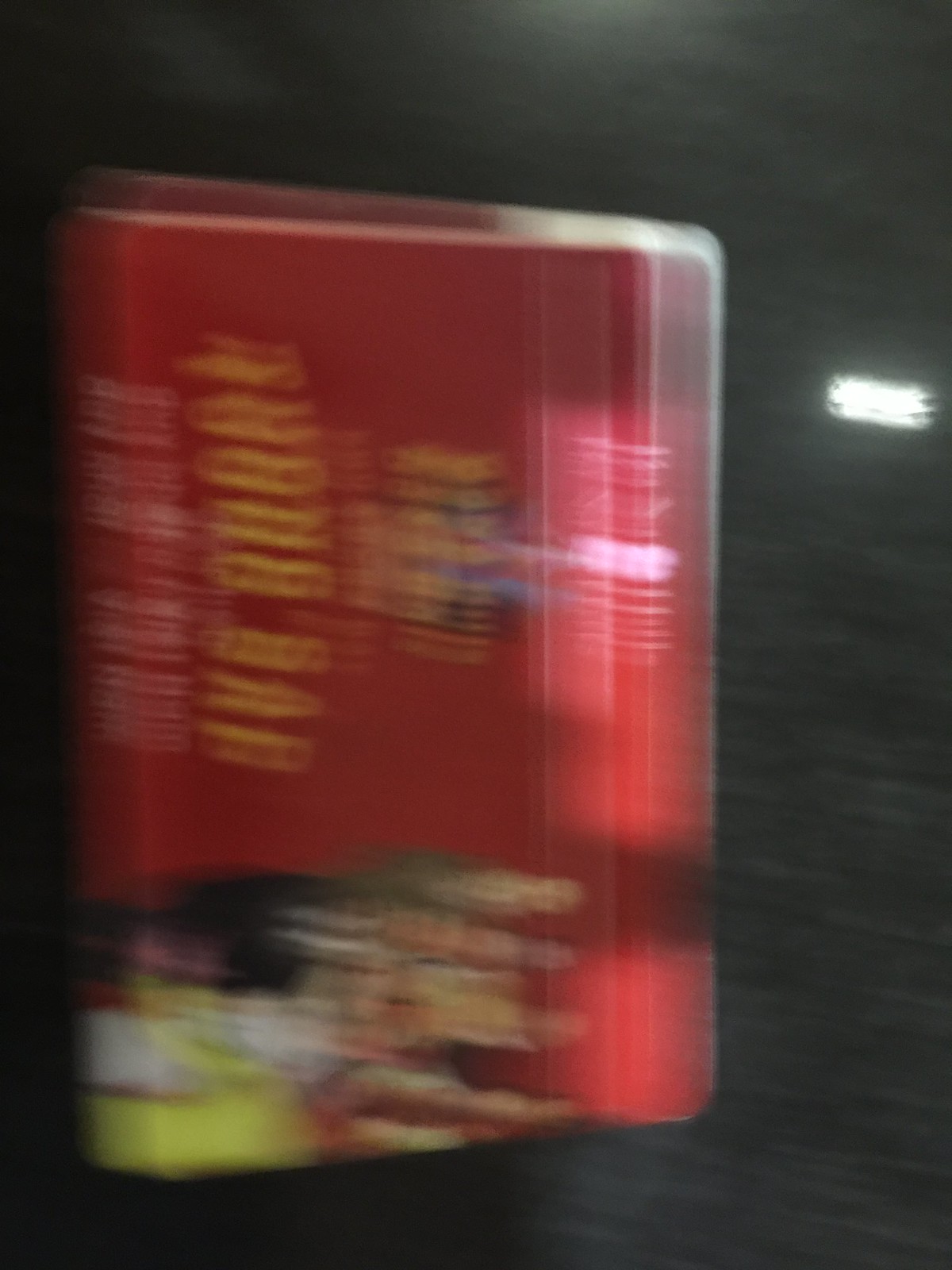A very blurry image depicts a red carton, possibly containing food, resting on its left side. The front of the carton, although facing the camera, is tilted with the bottom side pointing left. The carton features a white edging and appears to be open, providing a glimpse of its contents. Despite the blur, one can discern a group of people pictured on the side of the carton that is resting beneath it, while the product name is prominently displayed in yellow text at the upper part of the box.